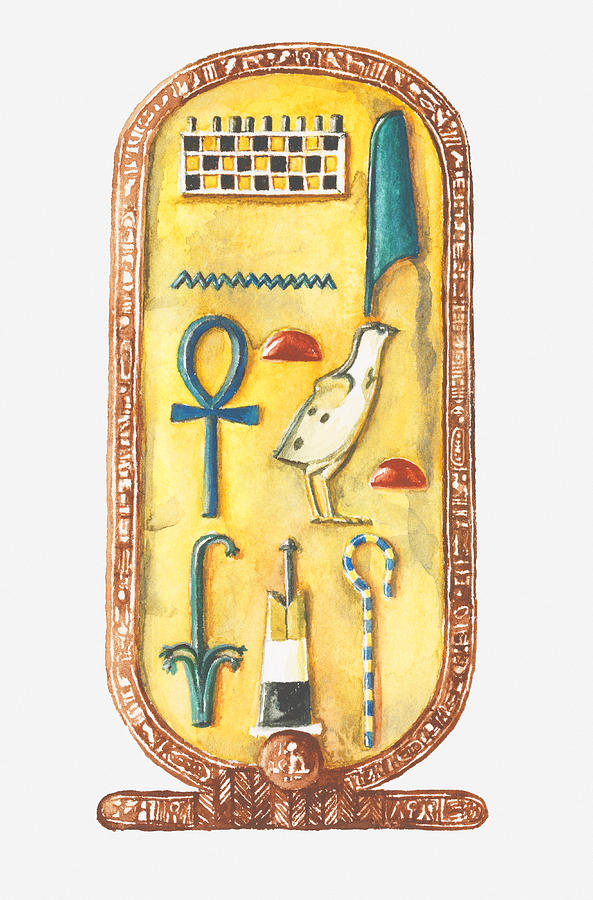The illustration depicts an ancient Egyptian hieroglyphic plaque. The plaque is long and oval-shaped with a base resembling a stand-up mirror. The frame of the plaque is a rusty brown color, adorned with white hieroglyphic writing. The interior is yellow. At the top, there is a black and yellow checkerboard pattern. To the right of this pattern is a teal green flag-like drape. Below the flag, there is a detailed bird, identified as a ptarmigan, with white feathers, a gray breast, two long legs, a short wing, a black crown, and dark polka dots on the backs of its wings. Next to the bird is the Egyptian Ankh symbol, A-N-K-H, in the same teal green color. Beneath the Ankh symbol, there's a simplistic flower, also in teal. Adjacent to the flower is an object with black, white, and yellow stripes, notched at the top with little antenna-like projections. To its right is a blue and yellow staff with a circular, crook-like top, reminiscent of a pharaoh's cane, which curves like a candy cane and has a section resembling a snake. The plaque's detailed design is evocative of Egyptian artistry and symbolism.